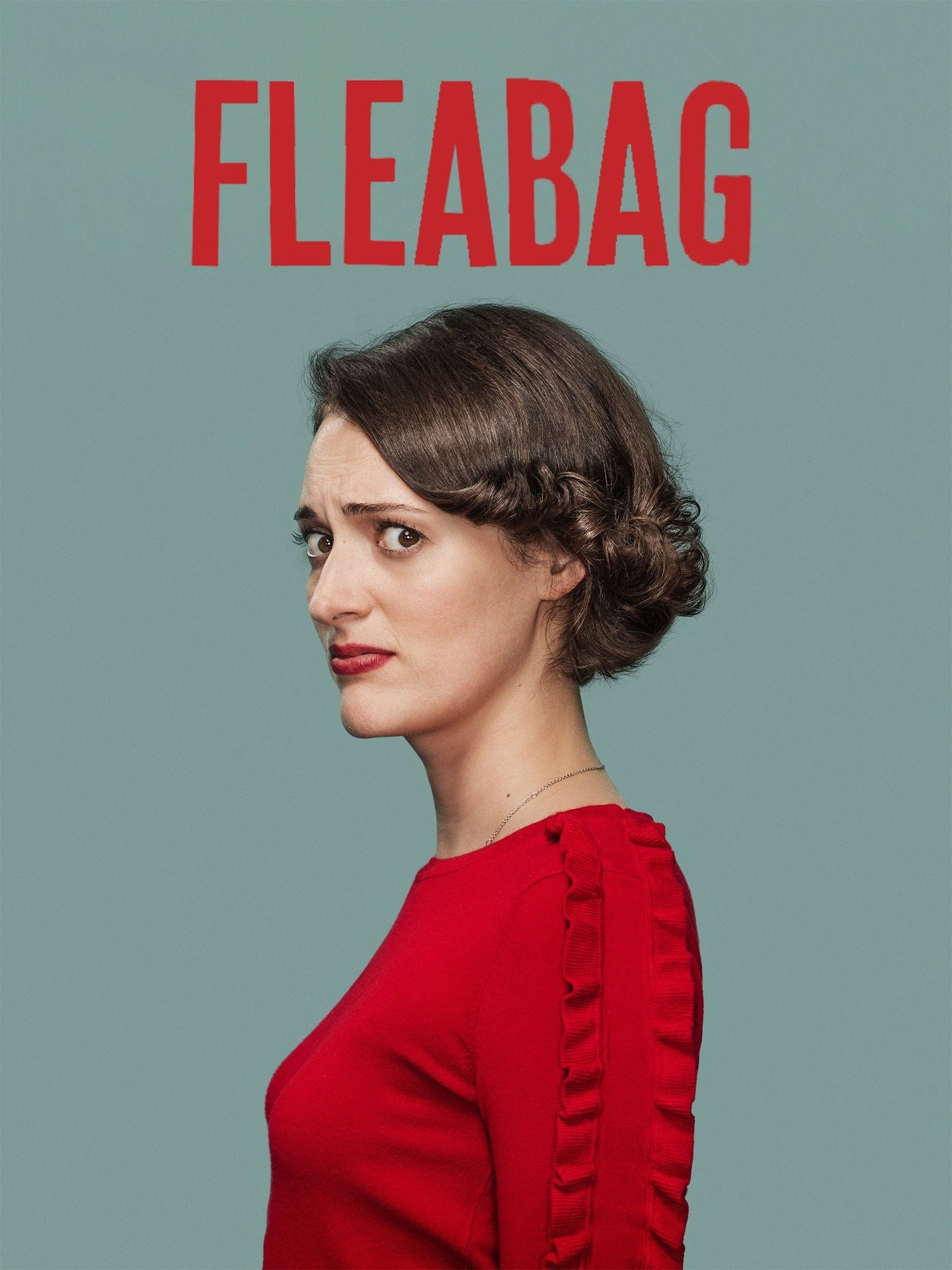The promotional poster for the television show "Fleabag" features a portrait of the actress Phoebe Waller-Bridge against a light teal green background. Prominently displayed at the top in bold, bright red uppercase letters is the show's title, "FLEABAG." Phoebe Waller-Bridge, positioned in the right profile, gazes towards the camera with a slightly wary expression, her eyes catching the viewer's attention. 

She has short, curly brown hair that reaches down to the nape of her neck, partially covering her ear. Her lips are adorned with red lipstick that matches her red outfit, which appears to be either a dress or a sweater. The outfit is detailed with ruffled fabric that runs from her neck down to her elbows, emphasizing the sleeve's design. A thin gold necklace is also visible around her neck. The overall photographic style of the poster is representational realism, capturing a detailed and authentic portrayal of the actress.